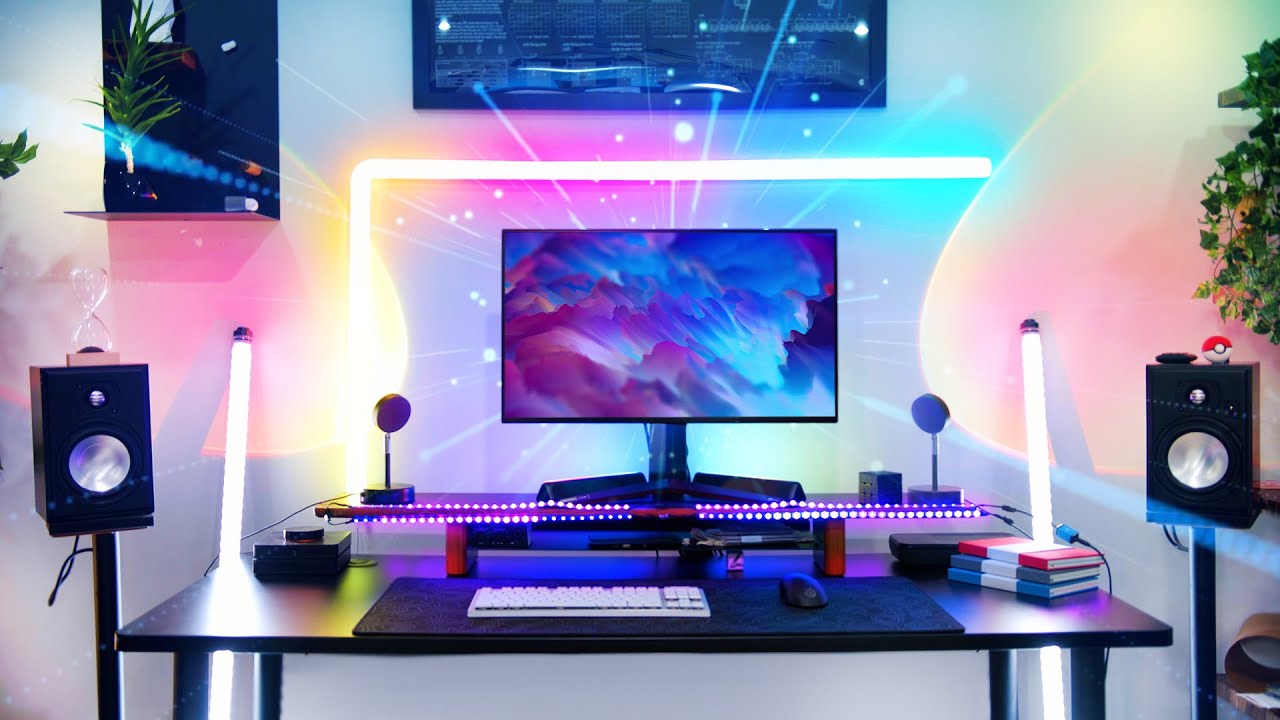This detailed digital art illustration showcases a futuristic and vibrant computer desk setup against a white wall adorned with plants and shelves. The centerpiece is a sleek black desk with a large 32-inch monitor on a riser shelf, surrounded by an array of LED lights. These LEDs illuminate the scene in a captivating rainbow color scheme of blues, pinks, purples, and yellows, creating a dynamic and lively atmosphere.

Two black speakers with silver cones stand on either side of the desk, complemented by smaller speakers and additional tubular LEDs integrated through the desk and its legs. On the right speaker sits a vivid red and white Pokémon ball, while the left features a clear hourglass. The desktop itself is organized with a black mat, a black mouse, a silver keyboard, and a stack of books—a red book on top of a green one, which in turn rests on a blue book.

Above the monitor, a neon light transitions from yellow on the left to pink and green on the right, further enhancing the futuristic aesthetic. Additional details include a black poster partly visible at the top middle and a black shelf holding a plant, contributing to the cozy yet high-tech ambiance suited for a gamer or a YouTuber.